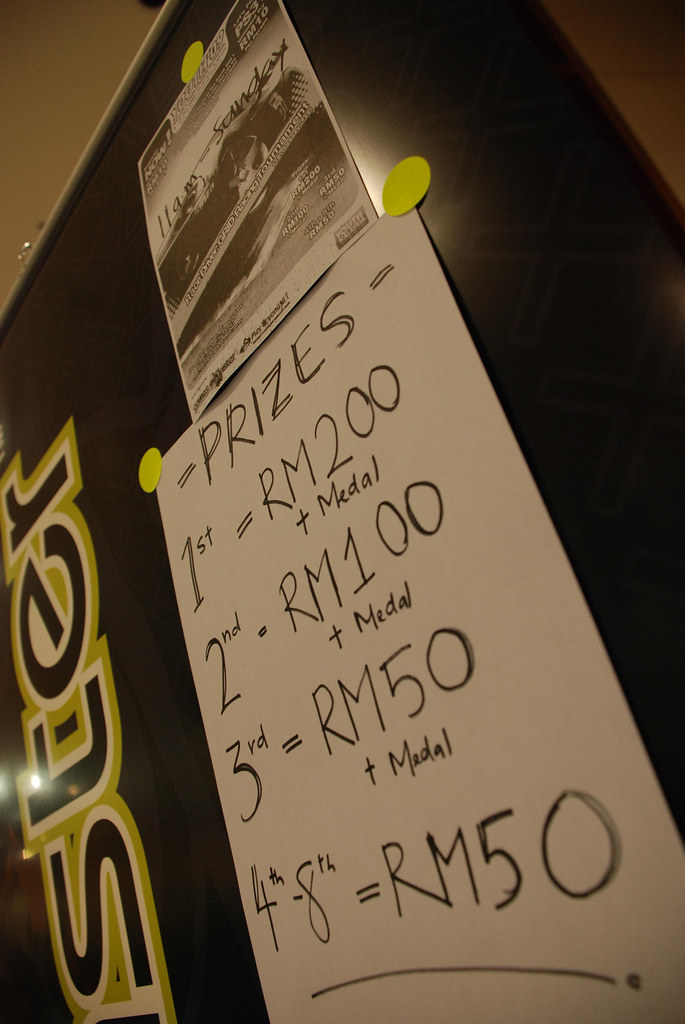The image depicts a black bulletin board with two pieces of paper affixed to it using circular yellow magnets. The top paper is a smaller, illegible flyer, while the larger sheet below is a handwritten sign on white paper with a black border and writing. The main sign provides detailed information about prizes, noting in black marker: "Prizes - 1st: 200 RM and a medal, 2nd: 100 RM and a medal, 3rd: 50 RM and a medal, 4th-8th: 50 RM." The board is positioned such that the ceiling with its lighter brown hue is visible above it. The setup is fairly plain with no added decoration, focusing solely on conveying the factual details of the contest rewards.